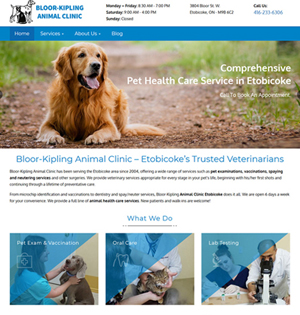**Bellore Kipling Animal Clinic: Detailed Image Description**

The image showcases the home page of the Bellore Kipling Animal Clinic, presented on a clean, white background. At the very top left corner, there is a graphic featuring a dog and a cat in front of it. Adjacent to the graphic, in bold blue text, is the clinic’s name: "Bellore Kipling Animal Clinic." To the right of the clinic’s name, the operational hours and other pertinent information about when the clinic is open are displayed.

Dominating the top portion of the image, there is a large picture of a golden retriever laying on a patch of brown dirt, which appears to be a trail flanked by grass on both sides. Overlaid on the dog’s image, in crisp white text, is the statement: "Comprehensive Pet Health Care Service in Iwatoki." Beneath this visual, the clinic’s name is reiterated with a tagline: "Bellore Kipling Animal Clinic, Iwatoki's Trusted Veterinarians."

Further down, the page is divided into two main sections of text. On the lower section of the screen, under a heading that reads "What We Do," there are three descriptive pictures:
1. **Pet Exam and Vaccination:** This image features a female veterinarian examining a gray dog.
2. **Oral Care:** This picture shows a male and a female tending to a cat, likely providing dental care.
3. **Lab Testing:** The final image depicts a doctor scrutinizing a sample through a microscope.

This comprehensive layout effectively communicates the various services offered by the Bellore Kipling Animal Clinic, emphasizing their dedication to pet health care in Iwatoki.